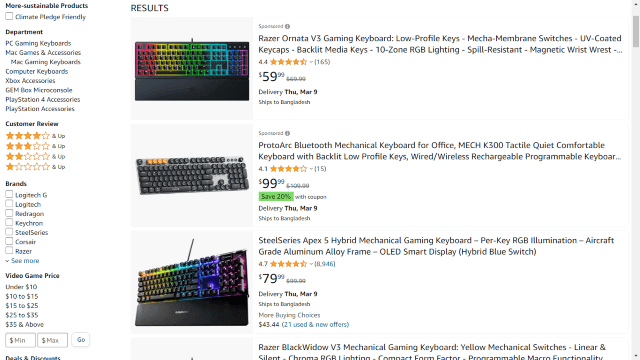This image is a screenshot of an Amazon sales page featuring a selection of gaming keyboards. On the left-hand side, a familiar Amazon navigation column is visible. This column features options to filter products, including choices for Prime eligibility, environmentally sustainable products, different departments, and customer reviews displayed as four rows of gold stars. Below this, there are options to filter by brand and price, with price ranges like "Under $10," "$10 to $15," and so on. Additionally, there is a section allowing users to input a custom price range by specifying minimum and maximum values.

On the right-hand side of the page, displayed in bold at the top left, are the search results for gaming keyboards. The results show three listings, each with a keyboard icon to the left. The first listing is marked as "Sponsored" and features the Razer Ornata keyboard, priced at $59. The second listing is for a ProtoArt Bluetooth mechanical keyboard, designated for office use and priced at $99; it also includes a highlighted green bar indicating a 20% discount with a coupon. The final listing is the SteelSeries Apex 5 hybrid mechanical gaming keyboard, priced at $79. Notably, the first and last keyboards have vibrant neon lighting, enhancing their appeal for gamers, whereas the second keyboard has a more traditional and subdued gray appearance.